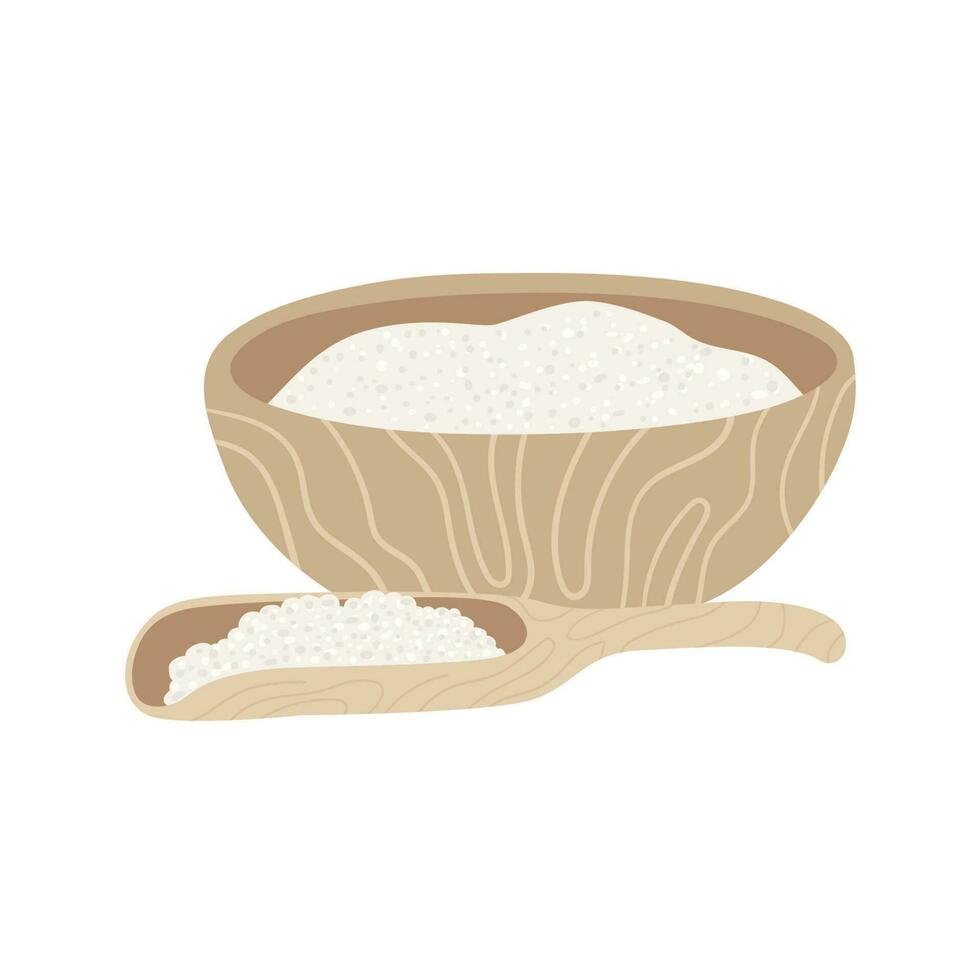The illustration features a brown, tan-colored bowl with abstract, self-design patterns resembling wood grain or topographical map lines. The bowl, light brown on the outside and darker brown on the inside, contains a mound of white, granulated, bead-like food, possibly resembling porridge, sugar, chia seeds, boba, or couscous. Each granule has white and light gray flecks. Beside the bowl, there is a matching spatula made from the same material, featuring similar wood grain-like structures. The scooper also contains a portion of the same white, bead-like food. The entire scene is set against a plain white background and styles as a clean, minimalist vector illustration focused on a food theme.